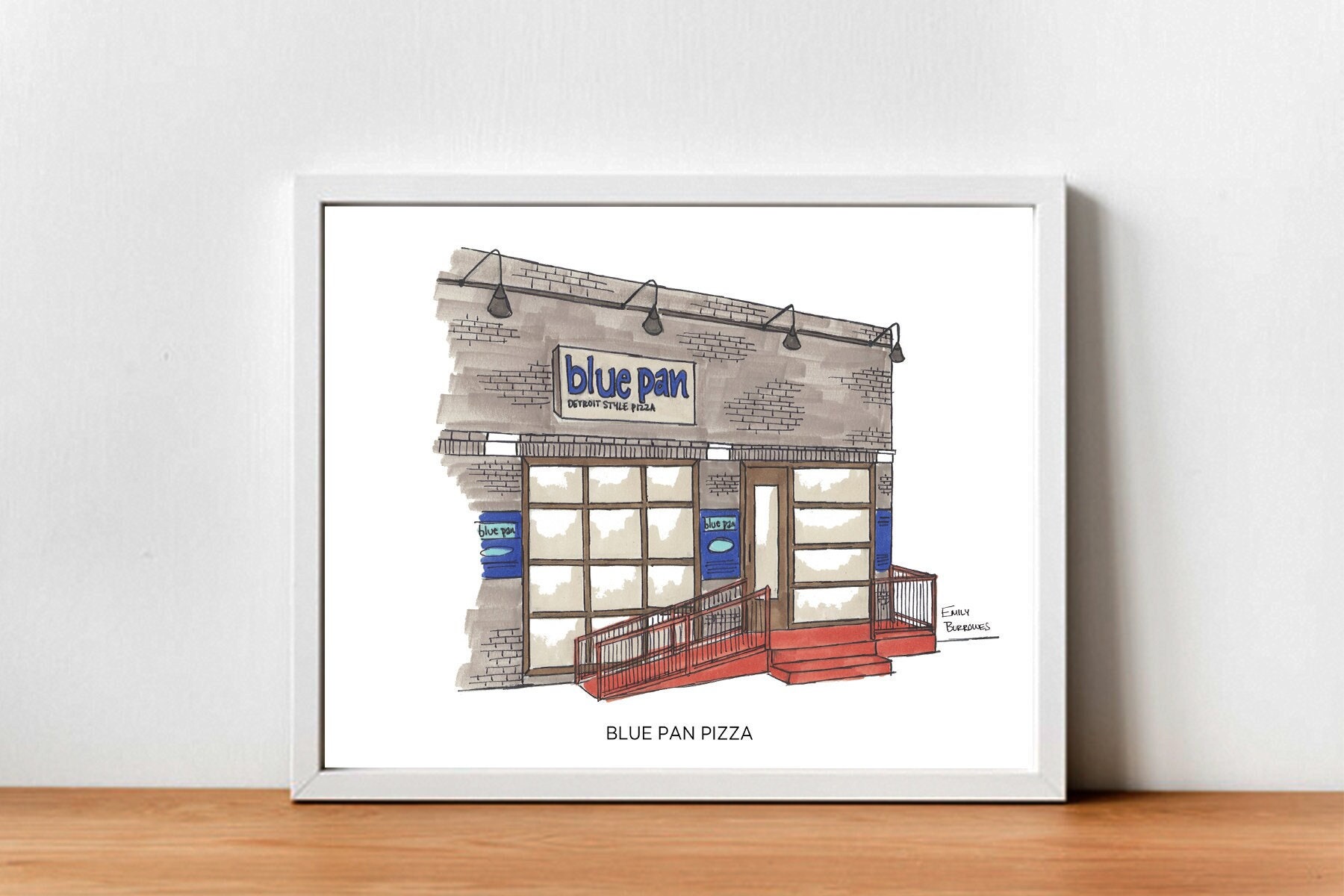The framed artwork depicted is a detailed watercolor rendering of a business named "Blue Pan Pizza." It features a prominent gray or white frame around it, and is set against a white background. The art itself captures a building with a distinctive gray brick wall. The centerpiece of the painting is the blue "Blue Pan" logo displayed in a light gray rectangle above the door. Below, in black typewritten letters, the caption reads "Blue Pan Pizza." The foreground includes red steps leading up to the entrance, which is a glass door with multiple panes, particularly noted are four horizontally oriented glass rectangles to the right of the door. The building facade showcases numerous windows with brown frames, contributing to the architectural detail. The rough edges of the watercolor strokes indicate the artist's technique, giving a dynamic texture to the piece. The artist's signature, "Emily Burroughs," is visible on the bottom right corner of the artwork. The artwork is displayed on a piece of wood, possibly a shelf, suggesting it is situated in front of the restaurant.